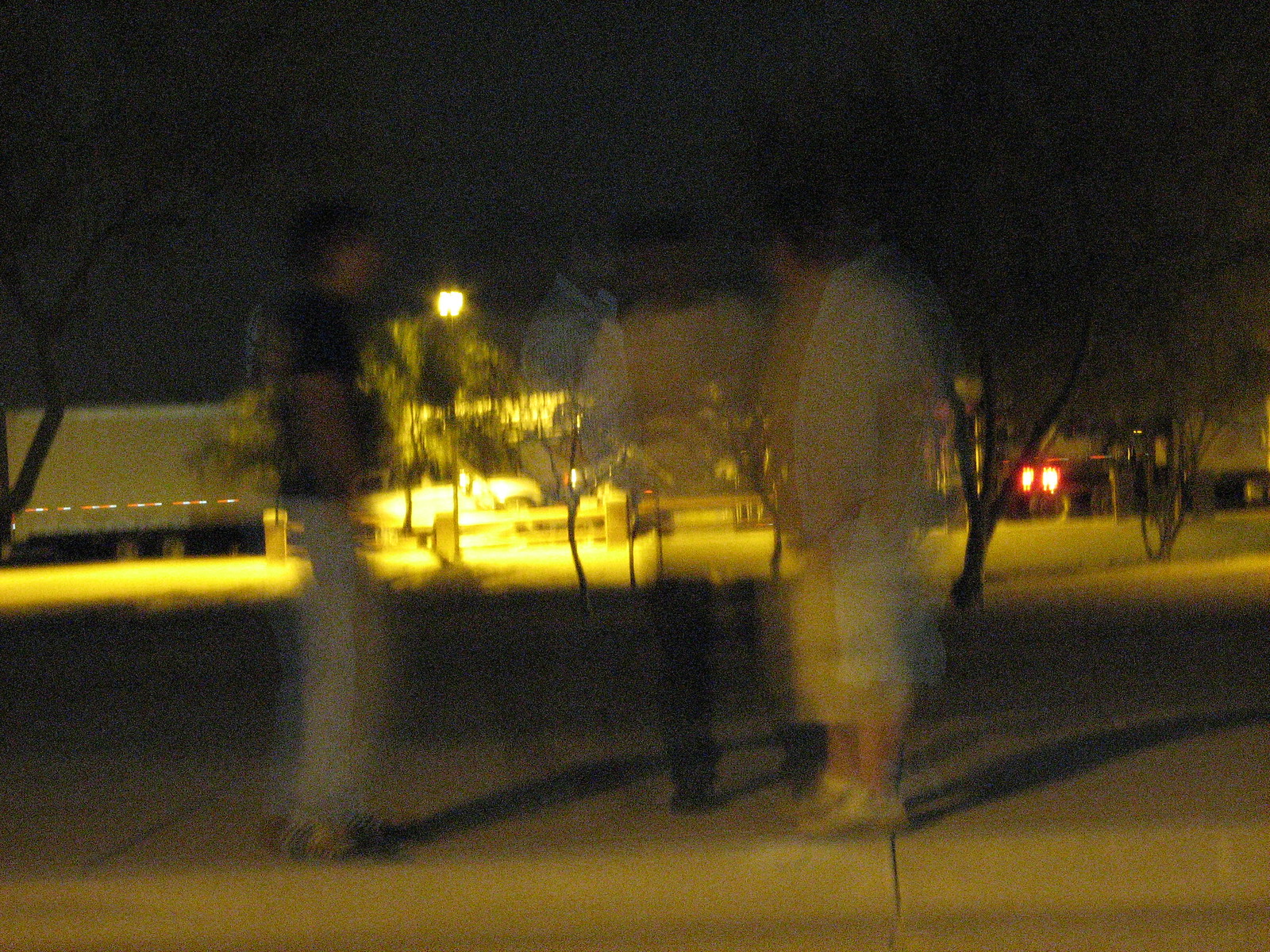This is a blurry and distorted color photograph taken at night, capturing the ethereal scene of three people standing around, appearing almost ghost-like. The image is illuminated by a yellow street light in the background, casting a warm glow over the area and creating long, black shadows that fall to the right. The person in the middle stands out particularly, as their blurred form lends an otherworldly, spectral quality. The individuals appear to be on a curbside lined with light gray concrete; one person wears light blue jeans and a short-sleeved black t-shirt, and another is dressed in a yellow undershirt with a white overshirt, shorts, and white shoes. There is discernible light gray road and a parking lot flanked by vehicles and semi-trailers to the left, with dark green-leaved trees surrounding the lot. Red lights are visible in the distant background, heightening the surreal and mysterious atmosphere of this nighttime scene.